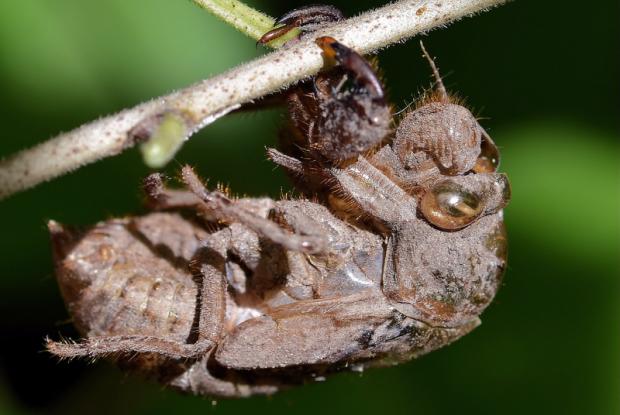This is a detailed close-up image of a dust-coated insect clinging upside down to a twig. The twig hosts a flower bud and possibly another leaf. The insect is not clearly identifiable due to being covered in dirt. Its coloration includes brown and tan, and its blurred eyes have a tan center with a hint of green. The insect appears to have brown claws and a possible stinger, suggesting it might be a wasp or bee. The background is an out-of-focus blend of green and black, potentially indicating grass and a shadowy tree. The overall tones of the image feature greens, blacks, whites, tans, and browns, but there are no other discernible objects or textures that confirm whether the setting is outdoors.